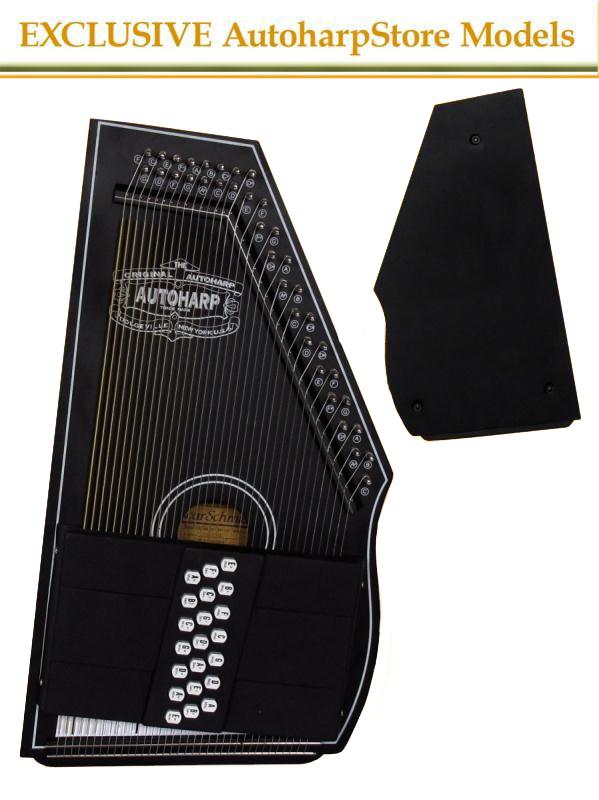This image appears to be an advertisement for exclusive models available at the Auto Harp Store. The ad features a white banner at the top, adorned with an olive-green and gold-colored line at the bottom. Centered in capital gold letters, it states "EXCLUSIVE AUTO HARP STORE MODELS."

The main focus of the image is a black auto harp, a stringed instrument reminiscent of a zither, but with more strings. The auto harp has a distinctive shape with a sharp angle on the right that leads the strings to progressively shorten from left to right, creating higher pitches. In the middle of the instrument, labeled "AUTO HARP," are numerous strings, possibly ranging from 10 to 30, and extending from long to short. 

Below this, the auto harp features white buttons that are likely labeled, though the text on them is unclear. The very bottom of the auto harp reveals more strings against a white background. Additionally, there's a notable, yet ambiguous, black object positioned to the right of the instrument, potentially a cover or another component, though its exact function is uncertain. The upper right part of the image also contains a completely black-filled outline of an auto harp, possibly representing the back side of the instrument.